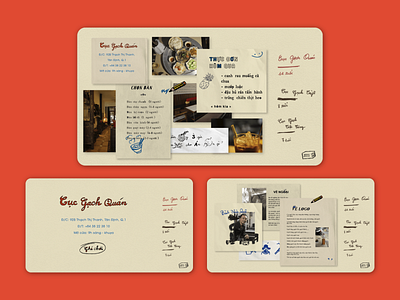The image displays three cream-colored recipe cards with rounded edges, arranged on a rusty deep orange, almost red background. The top card, larger than the other two, features small illustrations of food, drink, a pineapple, and a pencil. It is adorned with what appears to be various measurements and recipe details, along with layers of text that seem handwritten and include interior design sketches.

The bottom left card resembles a business card, showcasing red cursive text at the top and bottom, with finely printed blue text forming a list in the center. Some text on this card is circled, adding to its note-like appearance.

The bottom right card contains an assortment of pinned recipes and text, featuring a small image that looks like a microwave drawn in pencil, alongside more handwritten notes. This card also displays a photograph of a person, possibly the restaurant owner, accompanied by fragments of blue text and additional written content. The overall theme suggests these cards might relate to restaurant planning, featuring details like dish instructions, ingredient lists, and business information, though the exact text remains unclear due to the image quality.